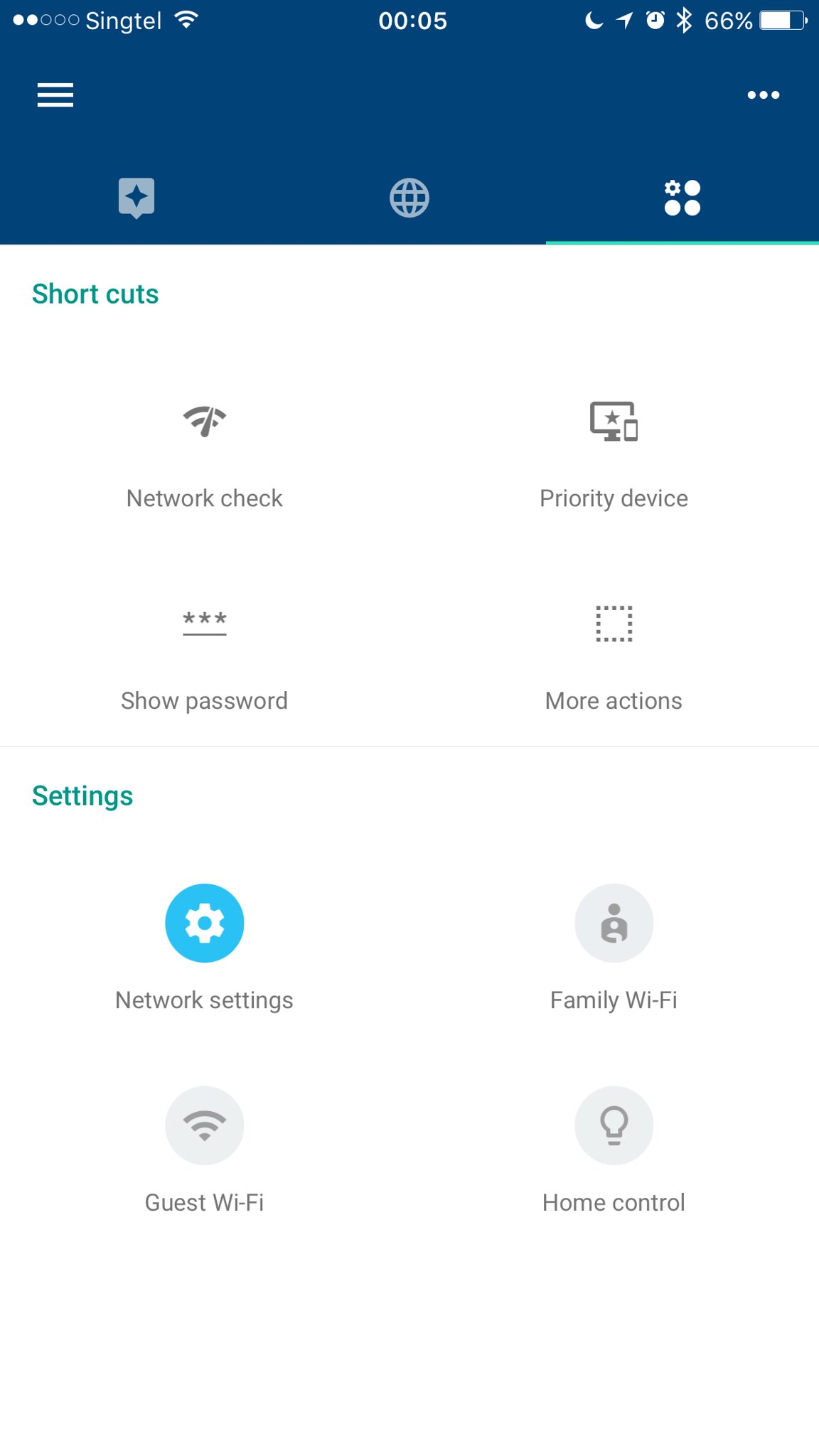Here is a detailed and cleaned-up caption for the image:

"A screen capture of a cell phone using the Singtel network, displaying a battery level at 66%. The screen shows the 'Shortcuts' section within the settings menu. Various shortcut options are visible, including 'Network Check,' 'Show Password,' 'Priority Device,' 'More Actions,' 'Settings,' 'Network Settings,' 'Family Wi-Fi,' 'Guest Wi-Fi,' and 'Home Control.' The interface features three navigation tabs at the top: the third tab is the current view, the second tab displays an icon resembling a globe, and the first tab has a diamond pattern icon. This screen is part of the settings where users can configure network and Wi-Fi options or manage home control settings."